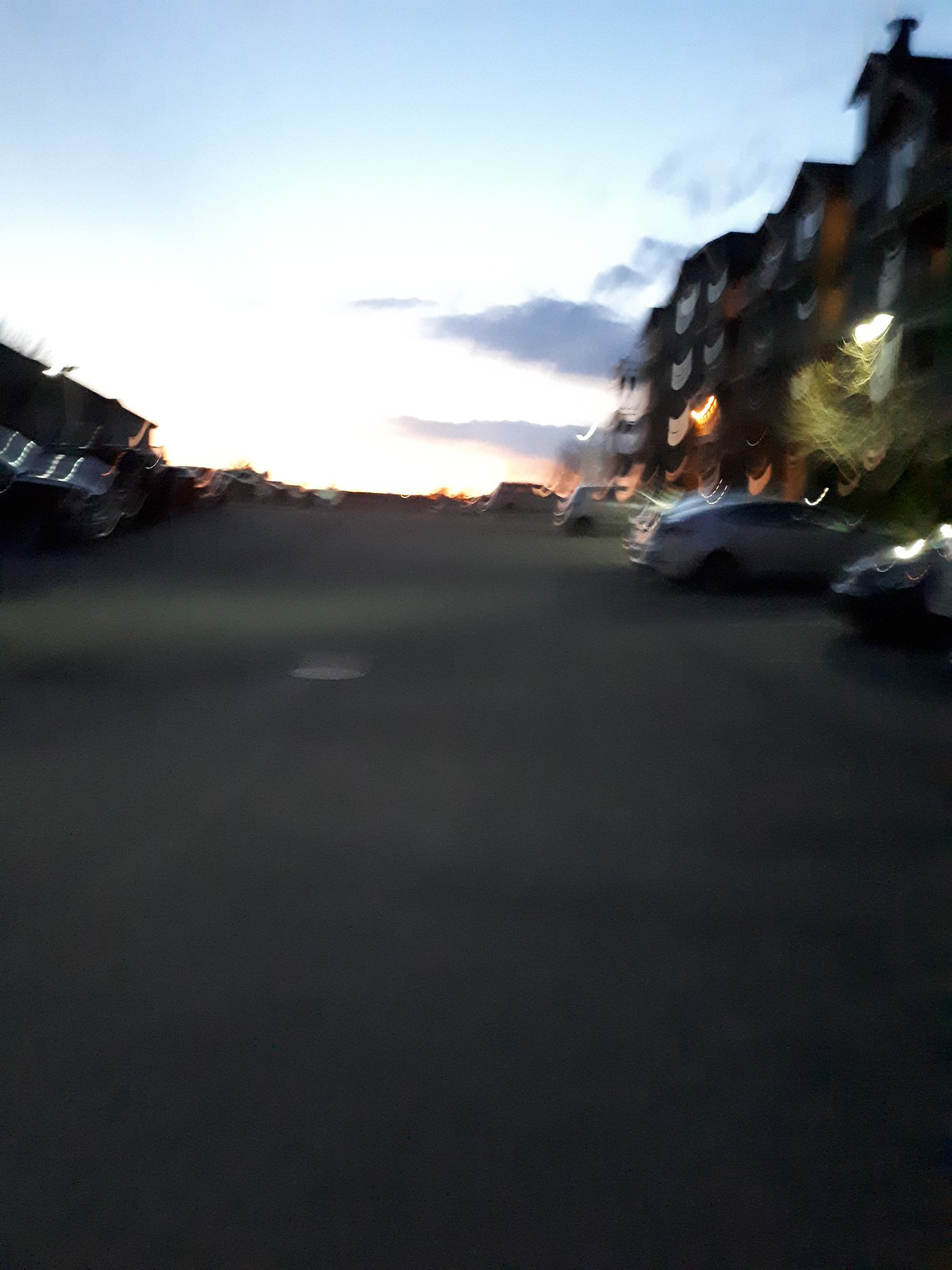This image depicts a large street scene taken during twilight, rendering the photograph somewhat blurry. The ground is composed of black concrete, indicating a well-used urban roadway. On one side of the street, several cars are parked adjacent to what appears to be a residential area, likely an apartment complex. Mirrors and windows reflect the ambient light that's dimming as dusk approaches. On the opposite side, more vehicles are lined up alongside a building, suggesting a densely populated area. The sky above is a mix of dusky blue and white, with thick, grayish-white clouds hinting at an overcast evening. The buildings in front of which the cars are parked are predominantly brown, contributing to a somewhat muted color palette that reflects the day's end.